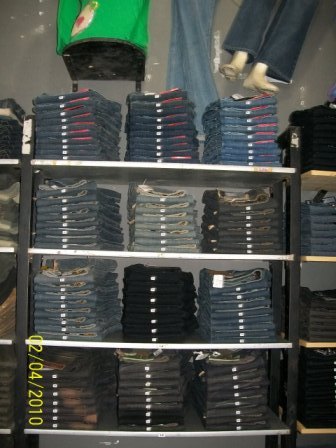The image depicts a neatly arranged display of jeans inside a department store. Multiple stacks of blue and black jeans are meticulously folded and placed on a four-shelf rack, commonly found in retail environments. Each shelf holds several neatly arranged piles of jeans, showcasing a variety of finishes, including light and dark denim. At the top of the display, the legs of a mannequin, dressed in jeans, are visible, suggesting it is attached to the wall above the rack. In the bottom left corner of the image, the date "02-04-2010" is vertically displayed in yellow. The overall scene is orderly, highlighting the organized presentation typical of store displays.